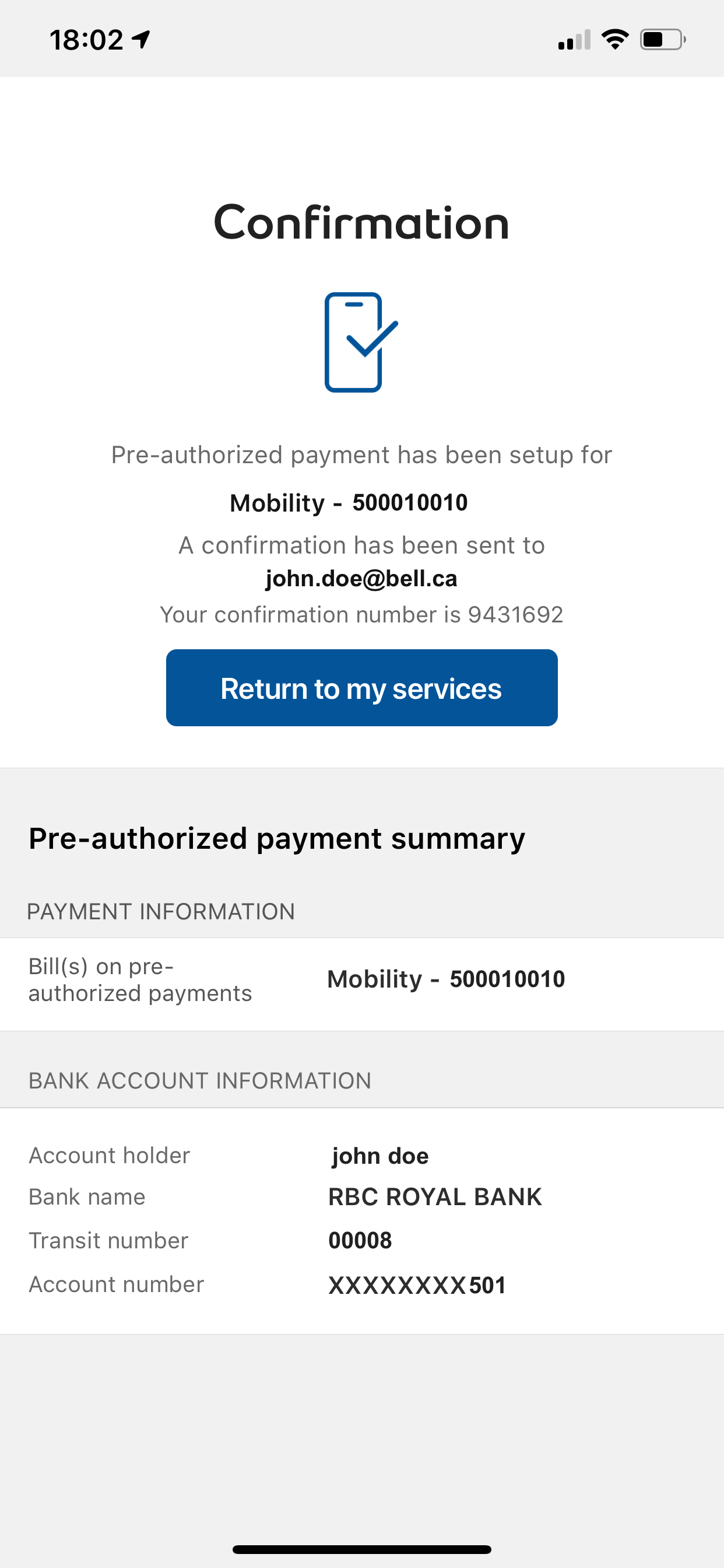Screenshot of a mobile app on an iOS device showing a confirmation screen for a pre-authorized payment setup. The time displayed is 18:02 with an active location tracker, 2 out of 4 cellular bars, a strong Wi-Fi signal, and approximately 45% battery life.

The main content of the screen includes a confirmation message with a small icon of a phone accompanied by a checkmark. The text reads:

"Pre-authorized payment has been set up for mobility-500010010. A confirmation has been sent to john.doe@bell.ca. The confirmation number is 9431692."

Beneath this message is a rectangular blue button labeled "Return to my services."

Following this button, a summary is provided:

"Pre-authorized Payment Summary: 
Payment Information: 
Bills on Pre-authorized Payments: Mobility-500010010

Bank Account Information:
Account Holder: John Doe
Bank Name: RBC Royal Bank
Transit Number: 00008
Account Number: XXXXXXXX501"